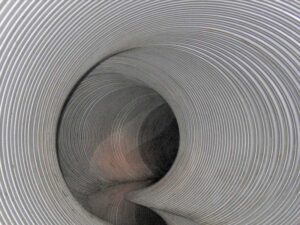The image features the interior of a large, curving tunnel that appears to be made of either metal or heavy-duty plastic material. The tunnel's walls are white with a ribbed or spiral design and it curves from the bottom middle of the image to the left and then back to the right. The tunnel floor has a reflective quality, suggesting the presence of water, and changes in color from a reddish brown near the entrance to a darker hue as it recedes into the distance. The tunnel's end plunges into darkness, enhancing the sense of depth and extending far beyond what is visible. The scene gives an impression of a sewer or drainage system, with a cylindrical, walkable passageway.